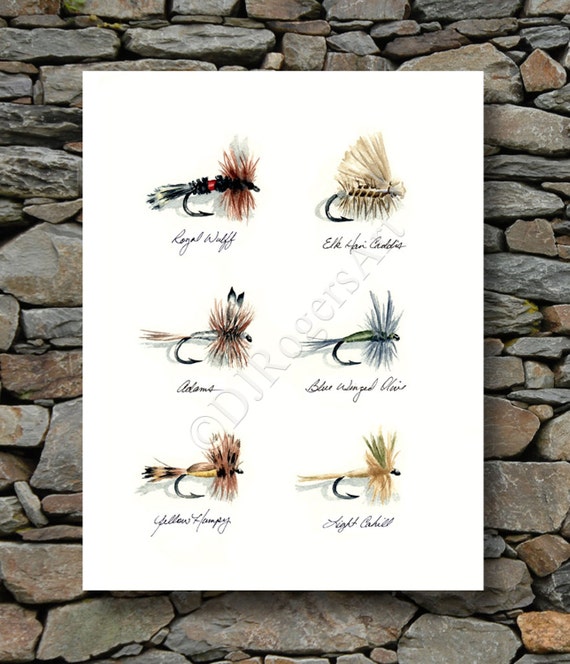This advertisement showcases six intricately designed fly fishing lures displayed on a large white poster board, set against a rustic stone wall made of varying pieces of shale and rock. Each lure has a distinct color and feather arrangement, accompanied by its name written in script, though somewhat hard to read. The lures are as follows: the top left is a Royal Wulff with a black hook and red and white feathers, next to it on the right is an Elk Hair Caddis featuring yellow and white hairs. On the second row, the left lure is an Adams, adorned with red and white hairs, while to its right is a Blue-Winged Olive, showcasing a green body and black and white hairs. The bottom row features a Yellow Humpy with yellow, red, and black feathers on the left, and a Light Cahill with yellow and green feathers on the right. The poster prominently displays the artist's signature, "D.J. Rogers Art," adding an element of craftsmanship to the visual presentation.